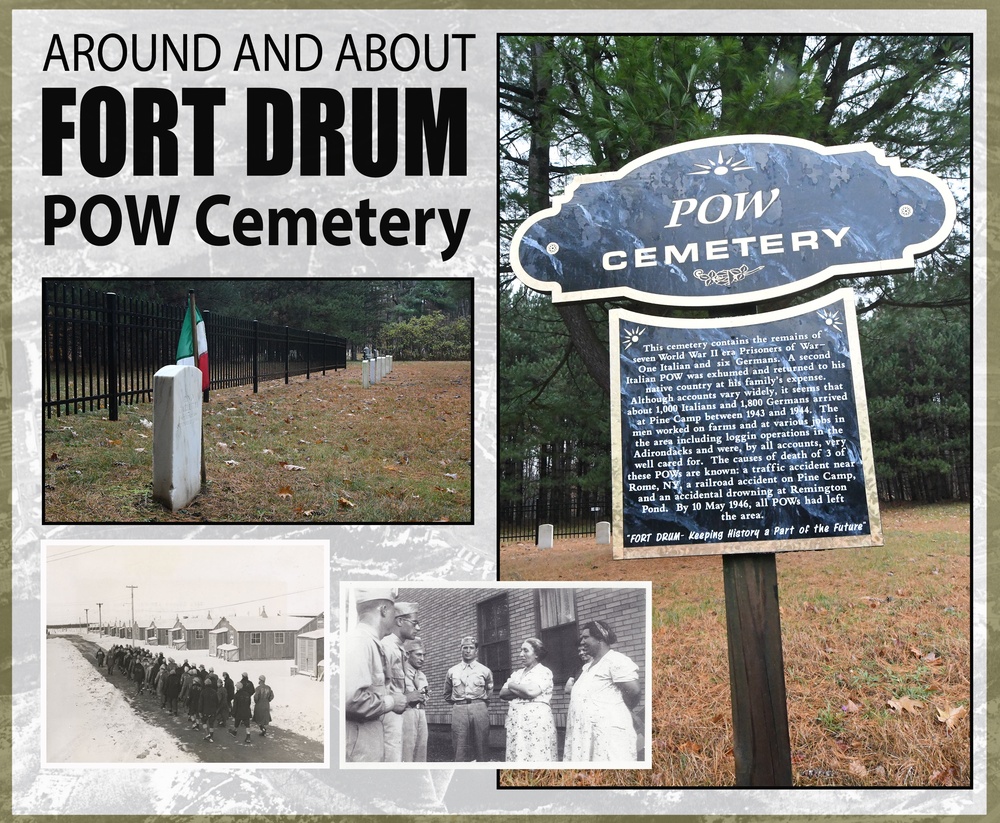The advertisement showcases the Fort Drum POW Cemetery, highlighting its importance and historical significance. At the top left corner of the ad, the text “Around and About Fort Drum POW Cemetery” is prominently displayed. The advertisement features a collection of images framed against a gold strip and a marbled gray background.

The first image beneath the text is a color photograph of a military gravestone, typically associated with a cemetery for prisoners of war. This headstone, set against an expanse of brown and green lawn and flanked by an iron black fence and a flag, stands as a solemn reminder of the lives commemorated.

Directly underneath, there is another black and white photograph depicting a crowd of people—likely soldiers and civilians—walking along a snow-covered path flanked by buildings and telephone poles, resembling a wartime scene either at a fort or barracks.

Next to it, another black and white photograph captures a moment among soldiers and three women. The women have varied expressions, with one looking skeptical, another contemplative, and the third faintly smiling.

On the right side, occupying half of the advertisement space, is a color photograph of a prominent sign within the cemetery grounds. The sign reads “POW Cemetery” and includes a detailed history of the cemetery, revealing that it holds the remains of seven World War II prisoners of war—one Italian and six Germans. It recounts the number of POWs who arrived at Pine Camp, now Fort Drum, and their activities, affirming that they were well-treated. The description ends with historical notes on the causes of death for three of the POWs and the eventual departure of all prisoners by May 10, 1946. The ad concludes with the phrase “Fort Drum, keeping history a part of the future,” emphasizing its commitment to historical preservation.